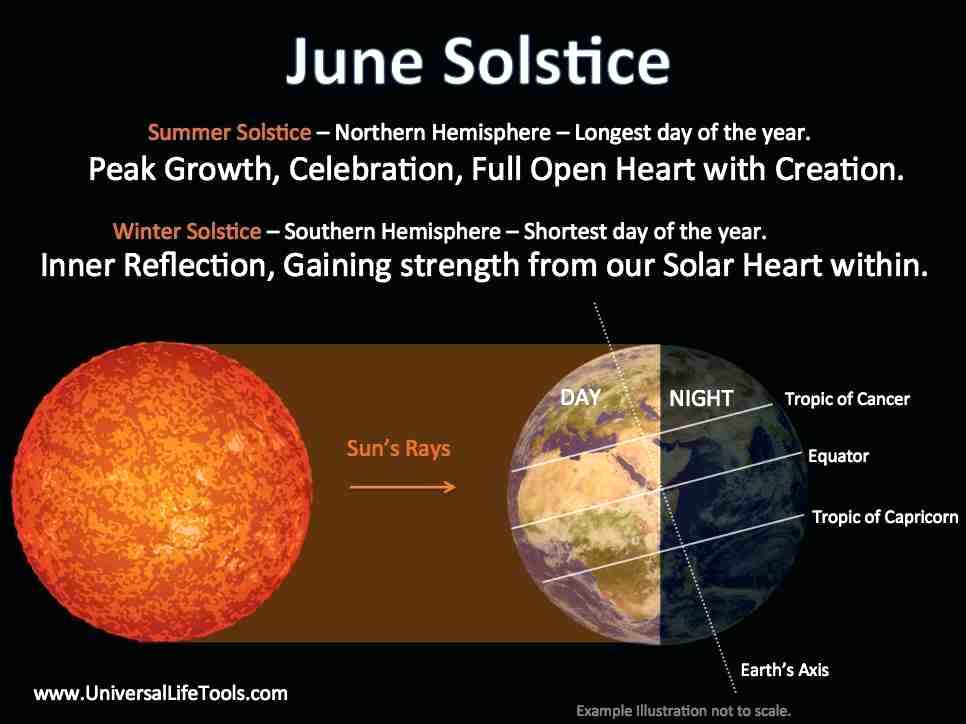The image features a black background with various informative texts and graphics about the June solstice. At the top, in white lettering, it reads "June Solstice." Below that, in dark reddish-orange text, it states "Summer Solstice – Northern Hemisphere – Longest Day of the Year." Further below, in larger white text, it says "Peak Growth, Celebration, Full Heart, Open Heart with Creation." Additional smaller text in orange-brown reads "Winter Solstice – Southern Hemisphere – Shortest Day of the Year," followed by "Inner Reflection, Gaining Strength from Our Solar Heart Within."

On the left side of the image, a close-up depiction of the sun is shown with a label "Sun Rays" in orange, accompanied by an arrow pointing towards the Earth. The Earth is illustrated as half illuminated (day) and half in darkness (night), with marked lines denoting the Tropic of Cancer, the Equator, and the Tropic of Capricorn. A diagonal line labeled "Earth's Axis" provides additional context. The bottom-left corner of the image includes the URL "www.universallifetools.com." This detailed visual and textual representation combines scientific information with philosophical reflections about the solstices.